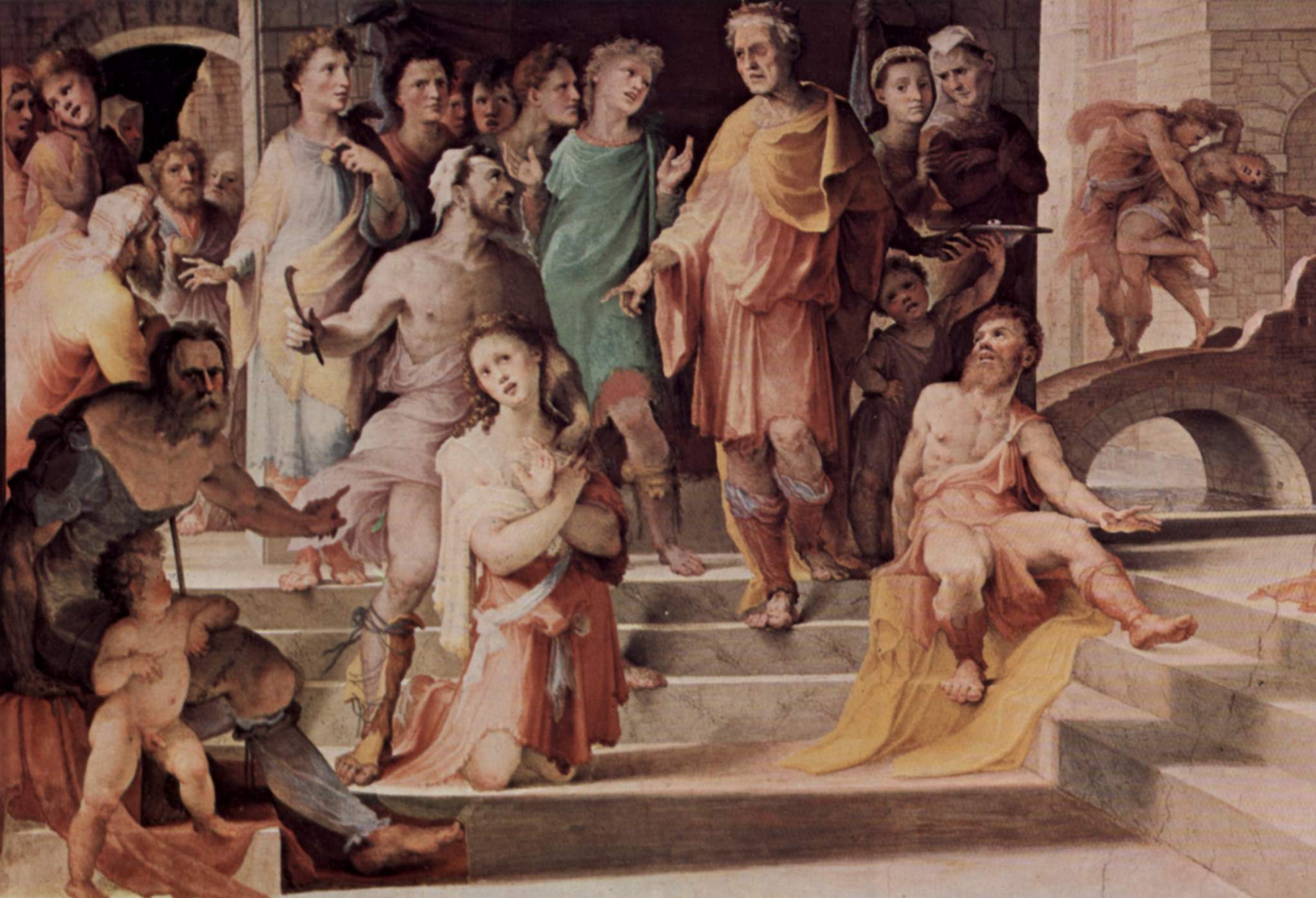This detailed photograph of an old, potentially religious painting centers around a significant Caucasian male figure positioned slightly to the right of center. This main character, possibly adorned with a crown and draped in fabric around his shoulders, wears knee-high shin guards. The scene unfolds on marble stairs with stone buildings in the background, suggesting an outdoor setting, as hinted by the observable daylight shadows.

Surrounding this central figure are approximately 20 individuals, all directing their attention towards him. Towards his bottom right, a man sits on the ground, gazing up, accompanied by a child. To the right of the scene, two cherub-like, angelic beings stand on a stone bridge. Additional figures include a nude baby located at the very bottom left and several women in the top left, appearing engaged in conversation but still focused on the central figure. 

The painting’s color palette is diverse, featuring hues of orange, black, gray, yellow, tan, green, black, brown, and hints of purple. The composition is dominated by the figures and the staircase ascending from the bottom center, creating a structured yet animated tableau within the overall room filled with people, devoid of any visible text.